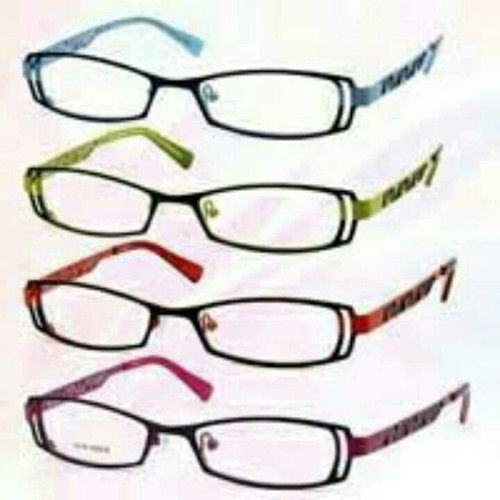This image showcases a promotional display of four pairs of eyeglasses, arranged vertically against a white background. Each pair features a black frame with arms and nose pieces in distinct colors. From top to bottom, the eyeglasses are blue, yellowish green, red, and purplish pink. Despite being positioned with some space between each pair, the overall picture lacks sharpness, appearing blurry and slightly enlarged. This setup highlights the different color options available for this particular eyeglass design, likely intended for advertisement purposes in a magazine or retail setting.